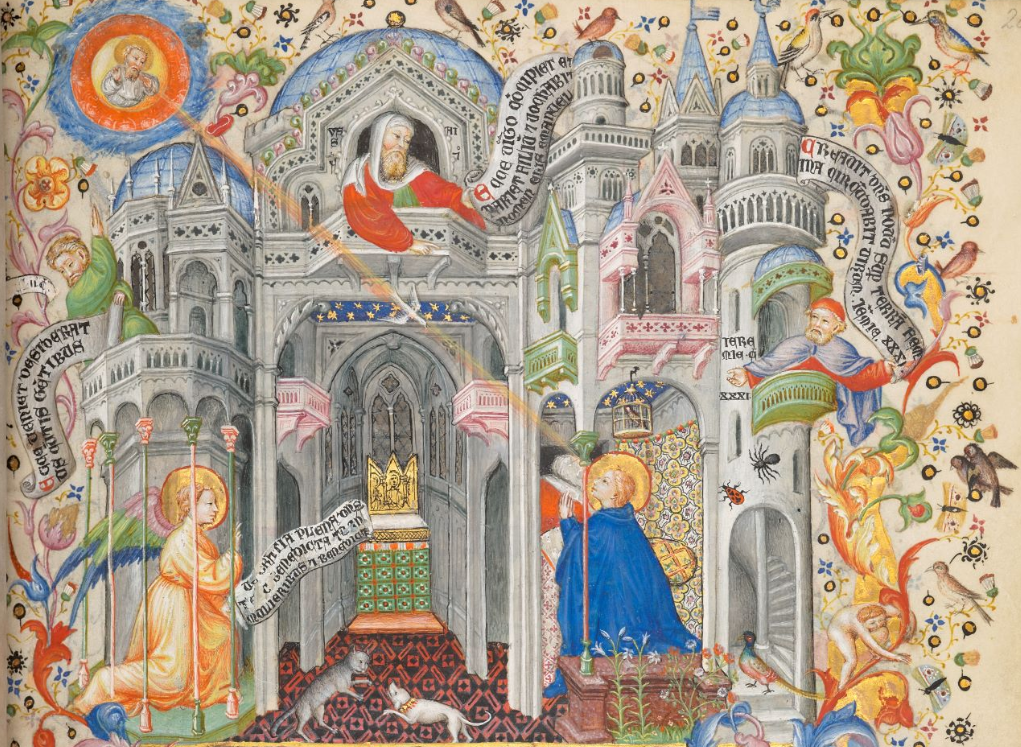This elaborate and colorful illustration, reminiscent of medieval and possibly Russian art, features an intricate depiction of a grand castle or religious building adorned with multiple elements. The central figure, standing on a prominent balcony, is an apparent holy figure dressed in red robes with a white head wrap, holding a long scroll that weaves through the right side of the image. Adjacent to him is another figure in a red gown and cap, also holding a banner with text. Below these figures are two angelic beings with vibrant wings and colorful robes—one in orange and the other in blue—kneeling and gazing upwards, suggesting a scene of devotion or reverence. At the base of the structure, a cat and a dog are present, adding a touch of earthly realism to the scene. Surrounding the castle is a visually rich array of intricate patterns featuring birds, butterflies, flowers, and various plants, which creates a lively and textured background. The illustration is a busy tableau of vivid hues—including pinks, greens, blues, reds, and whites—contributing to its almost mosaic-like quality, teeming with symbolic and ornate details.